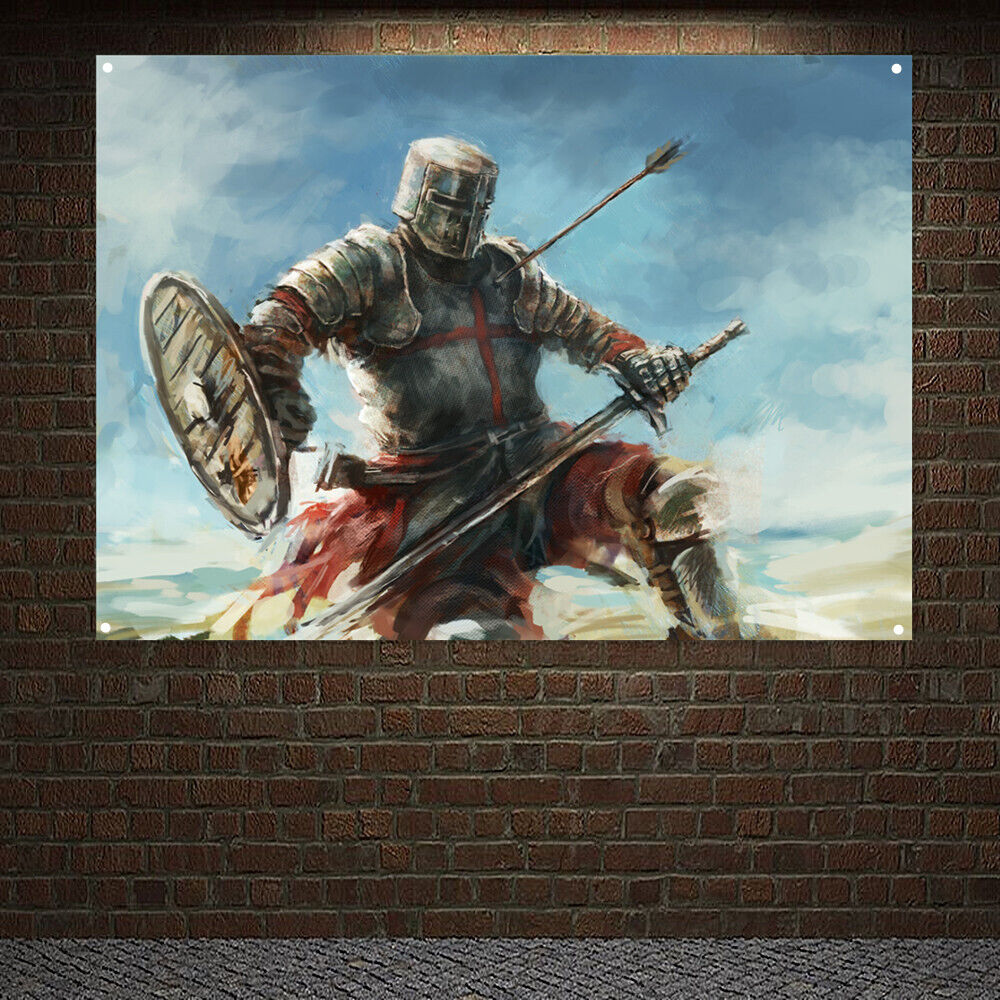This square outdoor image features a detailed photo of a landscape-oriented painting mounted on a brick wall. The wall, held together with concrete grout, displays the painting with visible fasteners at all four corners. Below the brick wall, a gray and black speckled sidewalk occupies roughly 5% of the image. The painting depicts a Crusader knight, clad in shining silver armor, riding a similarly armored horse. The knight's helmet has narrow slits for vision, and his gaze is directed slightly downward from the top left to the bottom right. He holds a long sword in his left hand and a shield adorned with a red cross in his right hand. The armor extends over his shoulders, chest, gauntlets, and down to his shins, with a belt around his waist supporting a sheath. An arrow pierces his left shoulder, suggesting he is in the midst of a battle. The background of the painting is a white sky interspersed with gray clouds, adding a somber tone to the scene. The Crusader's red cross emblem stands out against his silver armor, reinforcing his historical and religious significance.